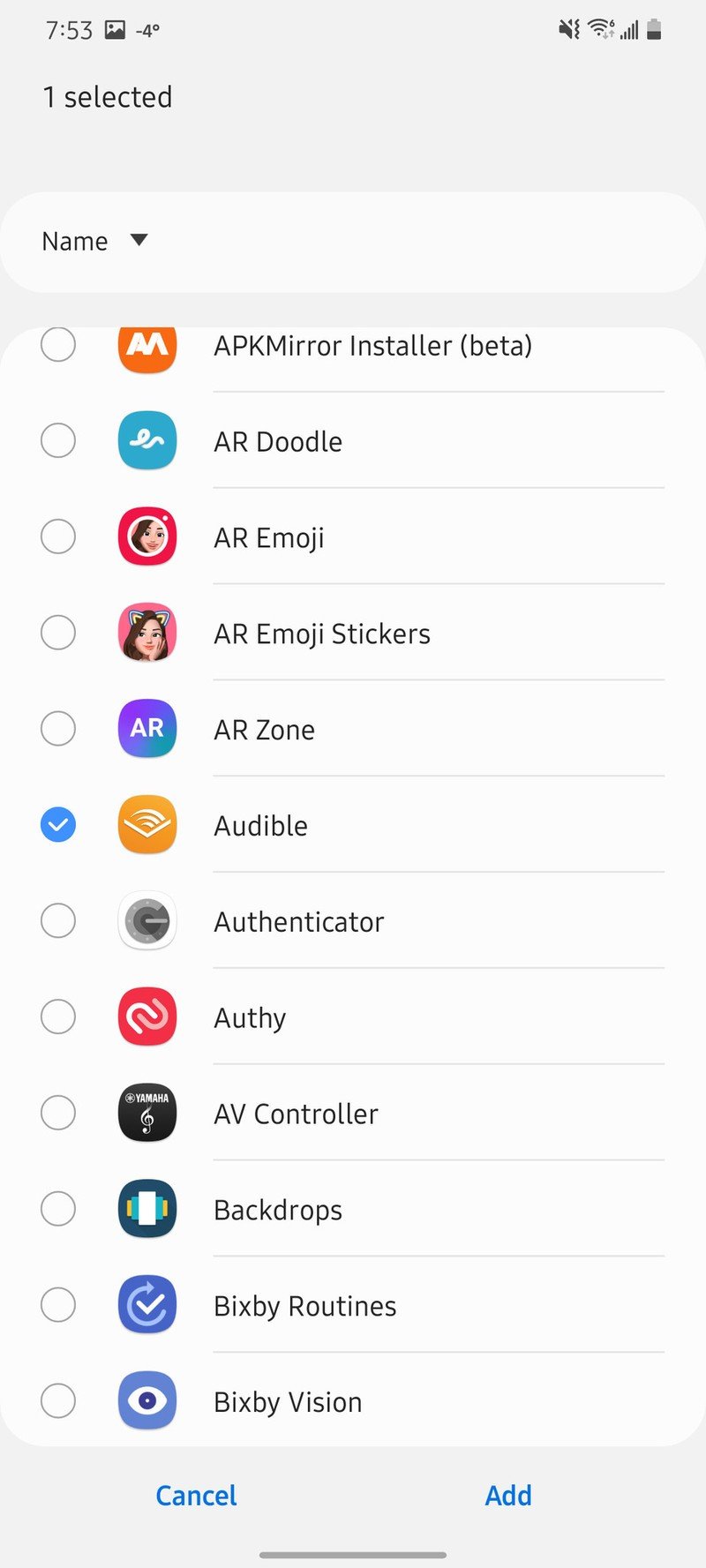In the image, there is a screenshot of a smartphone screen. At the top left corner, the time is displayed as 7:53. On the top right, several icons are visible: a screenshot icon, a temperature reading of -4 degrees, a battery icon, a network signal icon, a Wi-Fi 6 icon, and a mute icon. Below these icons, text reads "1 selected," which is positioned on the left side of the screen. Beneath this text, a drop-down menu includes application names.

A list of applications is displayed, including:

- APKMirror Installer (orange and white icon)
- Beta
- AR Doodle (blue and white icon)
- AR Emoji (pink and white icon)
- AR Emoji Sticker (pink icon with a cartoon picture)
- AR Zone (blue and white icon)
- Audible (highlighted, with a red and white icon, indicating "1 selected")
- Authenticator (white and grey icon)
- Albi
- AFV Controller (labeled Yamaha, black and grey icon)
- Backdrops (white, blue, and yellow icon)
- Bixby Routine (blue and white icon)
- Bixby Vision (blue and white icon)

At the bottom of the screen, there are two buttons, "Cancel" and "Add." Each application's distinctive icon and color scheme is noted, providing a clear and detailed description of the smartphone screen's content.